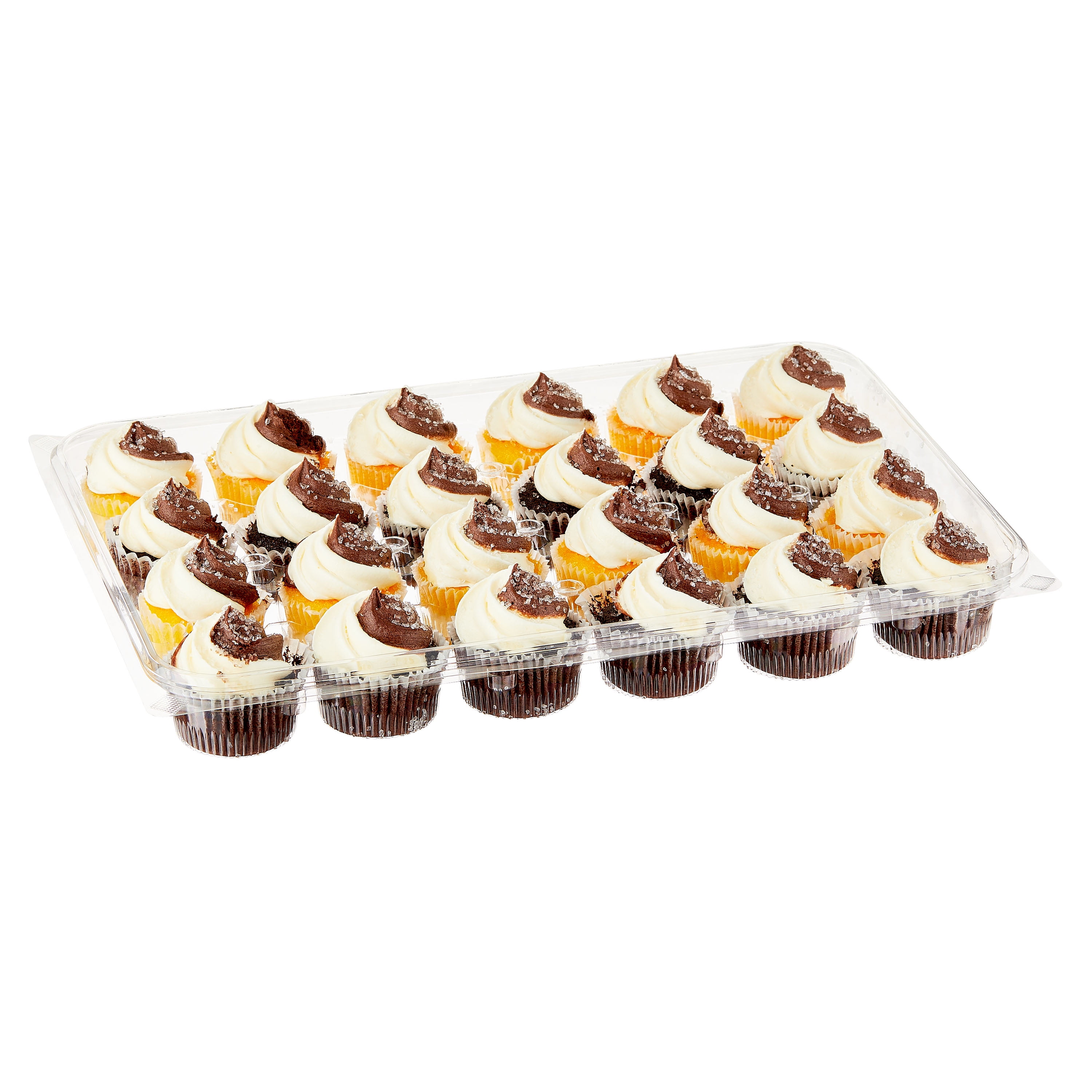This image features a rectangular, see-through plastic container holding 24 cupcakes arranged in six rows of four. Each cupcake sits in a white baking cup. The cupcakes alternate between chocolate and yellow (vanilla) cake. All of the cupcakes are topped with a creamy white frosting and a central dollop of chocolate. The clear plastic packaging is opened, displaying the detailed arrangement: the first row consists entirely of chocolate cupcakes with white frosting and a brown chocolate topping, followed by a row of vanilla cupcakes with identical frosting and topping. This pattern alternates throughout the container. The image is set against a white background, highlighting the contrast between the rich brown and yellow cupcakes, and their decorative frosting.